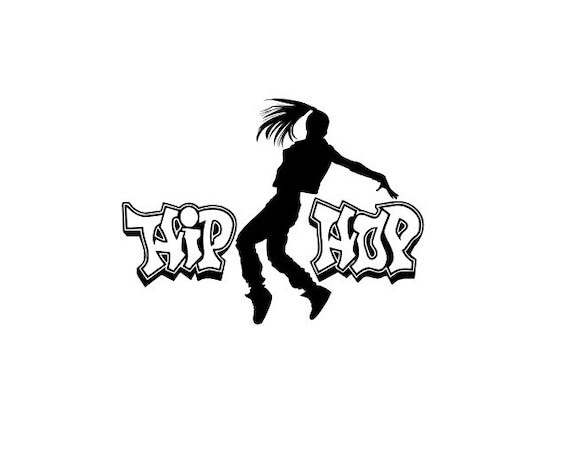This is a horizontal digital artwork set against a plain white background, featuring the stylized words "HIP HOP" in a graffiti-esque font. The words are rendered in white with a layered outline of alternating black and white, with additional thick shadows adding depth. Between "HIP" and "HOP" is the dynamic silhouette of a female figure mid-leap, suggesting a vibrant dance move. She is facing sideways to the left with her head turned toward the viewer, creating a sense of engagement. Her long ponytail fans out, emphasizing motion, and her left arm reaches out over the "P" in "HOP," almost touching it with her fingertips. She is depicted in baggy jeans, a jacket, and oversized shoes, further enhancing the hip-hop vibe. Her pose features bent knees and a twisted waist, as if she’s caught mid-spin or twist, capturing the essence of urban dance culture.